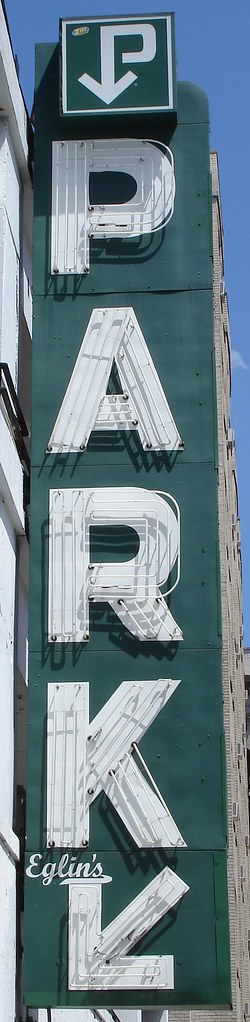The image depicts a tall, narrow, rectangular sign attached to a white building, typical for a parking garage. The sign is oriented vertically with the top outer edge rounded and has a dark green background. White lettering on the sign spells out "PARK" in descending order from top to bottom, beginning with the letter "P." Above these letters, in cursive white text, the word "Eglin's" is visible. At the very top of the sign, a white arrow is incorporated into a green square, forming a distinctive hook-like shape that points downward towards the letters below. Additionally, there's another white arrow pointing diagonally southwest, emphasizing the direction. A small portion of a blue sky provides a contrasting backdrop.